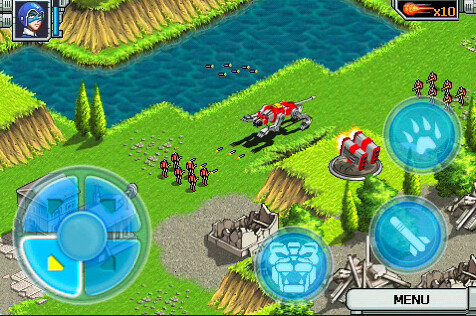The image showcases a vibrant video game screen set within a lush landscape featuring greenery, trees, and serene bodies of water. The scene appears to be from a world-building strategy game, where a tense battle unfolds: a mechanically engineered robot resembling a dog is engaged in combat with six characters armed with missile launchers. The display also includes an in-game menu and directional arrows, enabling players to navigate their characters across the terrain.